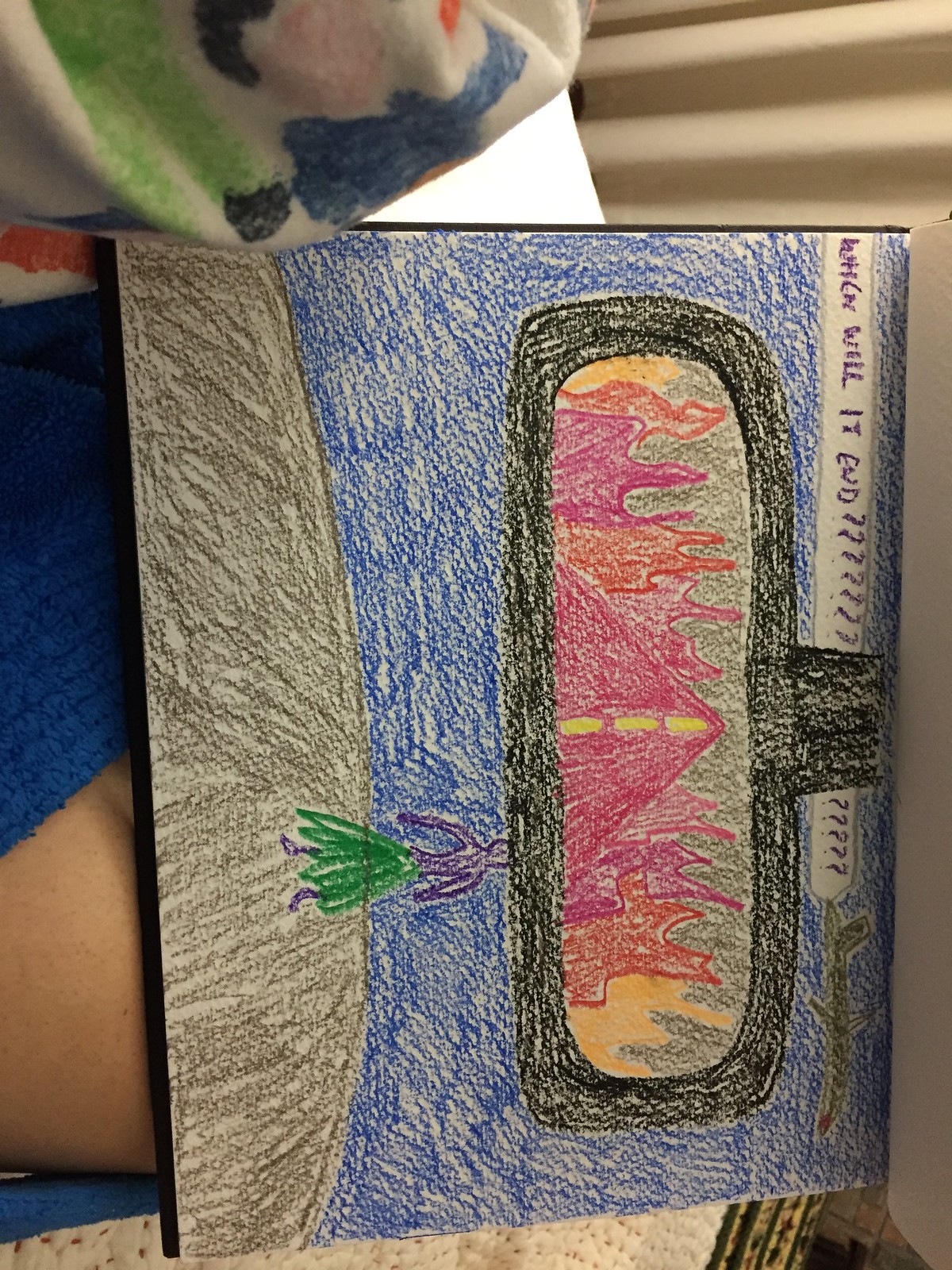The image is a child's colored drawing, depicted horizontally in a photograph. The drawing includes a perspective reminiscent of looking through a car's rear-view mirror. Surrounding the frame, the background is blue, representing the sky. At the top of the drawing, in purple text, are the words "When will it end," followed by numerous question marks.

Central to the image is the rear-view mirror itself, illustrated in black, showing a road with a reddish hue and a yellow dashed center line, flanked by orange, yellow, and reddish flames. This depiction suggests a sense of urgency or danger. In the foreground, near the bottom of the drawing, is a purple figure resembling a person or a figurine, dressed in a green skirt, possibly meant to resemble a hula skirt, standing on a brown or black surface that might be interpreted as the ground or dashboard.

In the photograph, the drawing is set against a lap covered by a blue short sleeve shirt, with the arm of the wearer visible and leaning on a blue object with white sidings underneath. Additionally, in the upper right of the actual photograph, there is a piece of cloth featuring green, blue, and black designs, adding context to the setting in which the drawing was photographed.